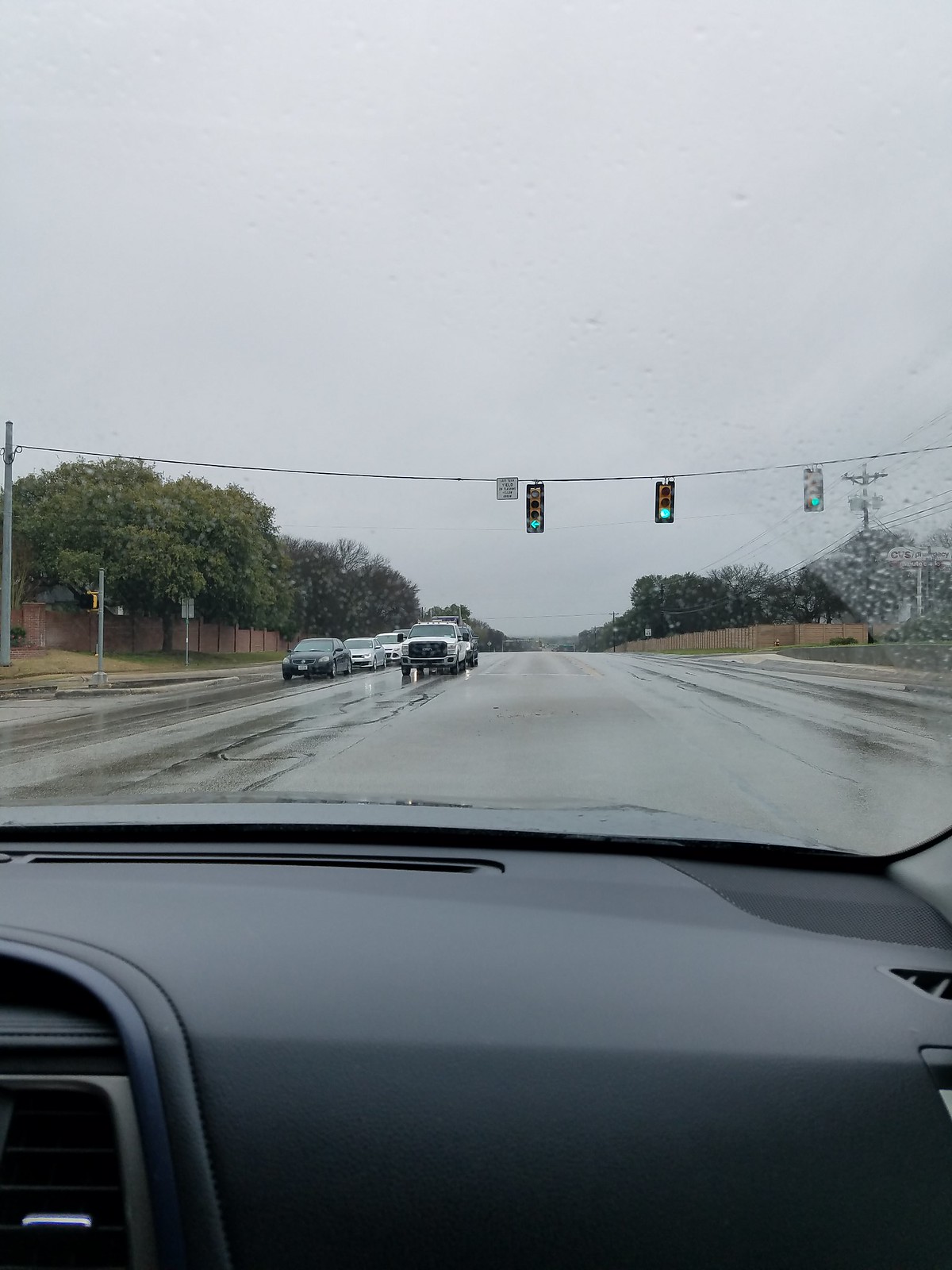A photo taken from the passenger side of a car captures a detailed view through the windshield, prominently displaying a section of the black dashboard. Ahead lies a multi-lane road; to the left, two lanes extend into the distance, filled with cars halted at a stoplight. Above, three green traffic lights dangle from a suspended wire, accompanied by a small white sign in the center of the wire. The road ahead glistens with moisture, evidence of recent rain, and is bordered by trees and a brown fence farther down. The overcast sky casts a gray hue over the scene, while raindrops are visible on the upper right corner of the windshield.